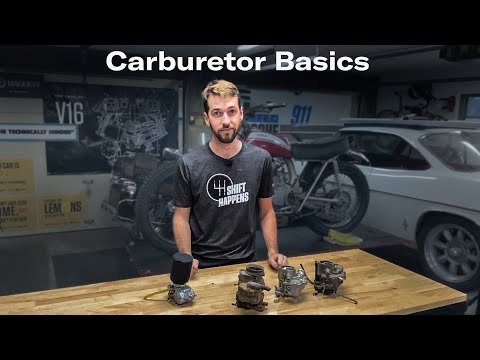In this color photograph or video freeze-frame, a man is depicted standing in a garage workshop. He appears to be around 30 years old with light brown hair and a full beard, wearing a dark gray shirt with the phrase "Shift Happens" and an illustration of a car shifter on it. The man is positioned behind a light beige wood table, upon which there are five carburetor parts displayed in a row. Each carburetor part is predominantly silver with dark brown and black elements, roughly the size of the man's hand. The setting features a professional and instructional atmosphere, enhanced by a white text headline above the man's head that reads "Carburetor Basics." In the background, a white sedan with a tire out and a motorcycle are visible, alongside various engine-themed posters, including one highlighting a V16 engine. The overall style of the image leans towards Photographic Representationalism with Realism, capturing a clear and detailed moment possibly linked to a tutorial or educational segment.